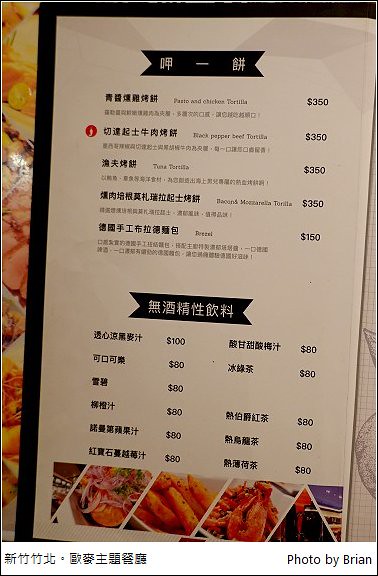This photograph captures the menu of a Chinese restaurant. The menu prominently displays various tortilla dishes at the top, listed as Pasta & Chicken Tortilla Pesto, Black Pepper Beef Tortilla, Tuna Tortilla, Matzo Mozzarella Tortilla, and an unreadable item, each priced at $3.50. The unclear pricing leads to potential confusion, as there is no decimal point between the numbers, making it appear as $350. The last unreadable item is listed at $1.50. The majority of the menu text is in Chinese. 

The lower section of the menu features prices organized in two columns: the left column has items priced at $100, $80, $80, $80, and $80, while the right column lists items all priced at $80. The menu itself is white with black banners and borders, and it's being held over a buffet table. 

At the bottom of the menu are images of various foods, including what appears to be crab and a salad, among other unidentifiable dishes. In the bottom right corner, there is a credit stating “Photo by Brian.”